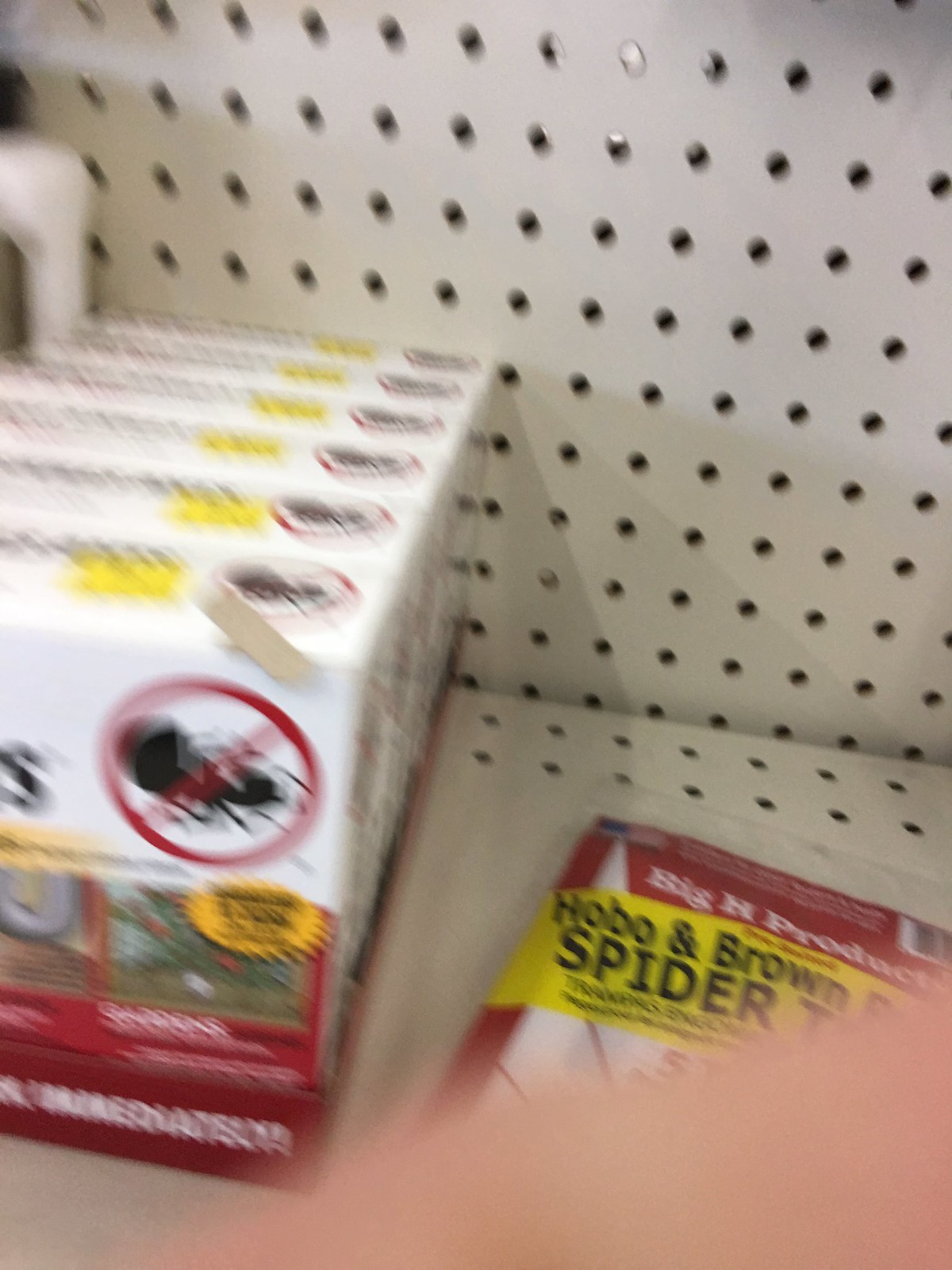A slightly out-of-focus image depicts a store shelf with a pegboard backing prominently visible. On the shelf, there is a box containing seven white packages of an insecticide product. Each package features a distinctive emblem: a red circle with a line through it over a sketch of a dead insect, signifying its pest-control purpose. Adjacent to the insecticide, there is a single package laid out that mentions "hobo" and "brown spiders," suggesting it is a repellent specifically targeting those types of spiders. The assortment and arrangement of these items point towards a section dedicated to pest control solutions.